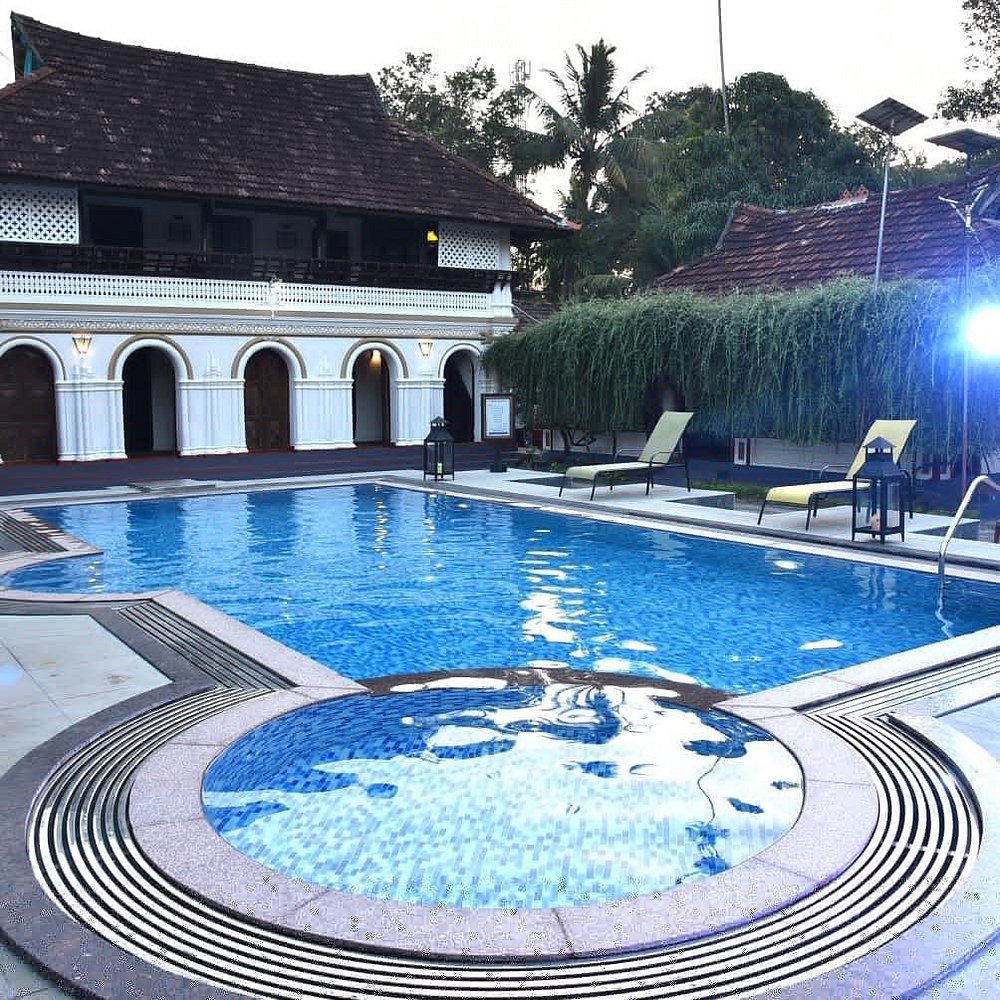This photograph showcases an elegant outdoor pool area set in a serene, lush environment. The main pool is rectangular with deep blue water, featuring a half-arch alcove on the left side. Dominating the bottom center of the image is a slightly elevated, round hot tub area with water gently overflowing its concrete rim, creating a visually pleasing effect. On the right side of the pool, about midway, there's a steel ladder for easy access. Positioned near the ladder are two inviting lounge chairs with vibrant yellow and green padding, accompanied by large glass and metal lanterns that hint at nighttime swimming.

Surrounding this tranquil setting is a trellis adorned with climbing vines and moss, backed by a shake roof barely visible through the dense foliage. In the background on the left side, a striking white villa with five archways and a second floor, also topped with a shake roof, adds a touch of architectural elegance. This structure gives the impression of a high-end hotel or a luxurious backyard retreat. Completing the scene are tall trees, including palm trees, that provide an additional layer of privacy and beauty. Overall, the image exudes a peaceful atmosphere, making it an ideal spot for relaxation and leisure.